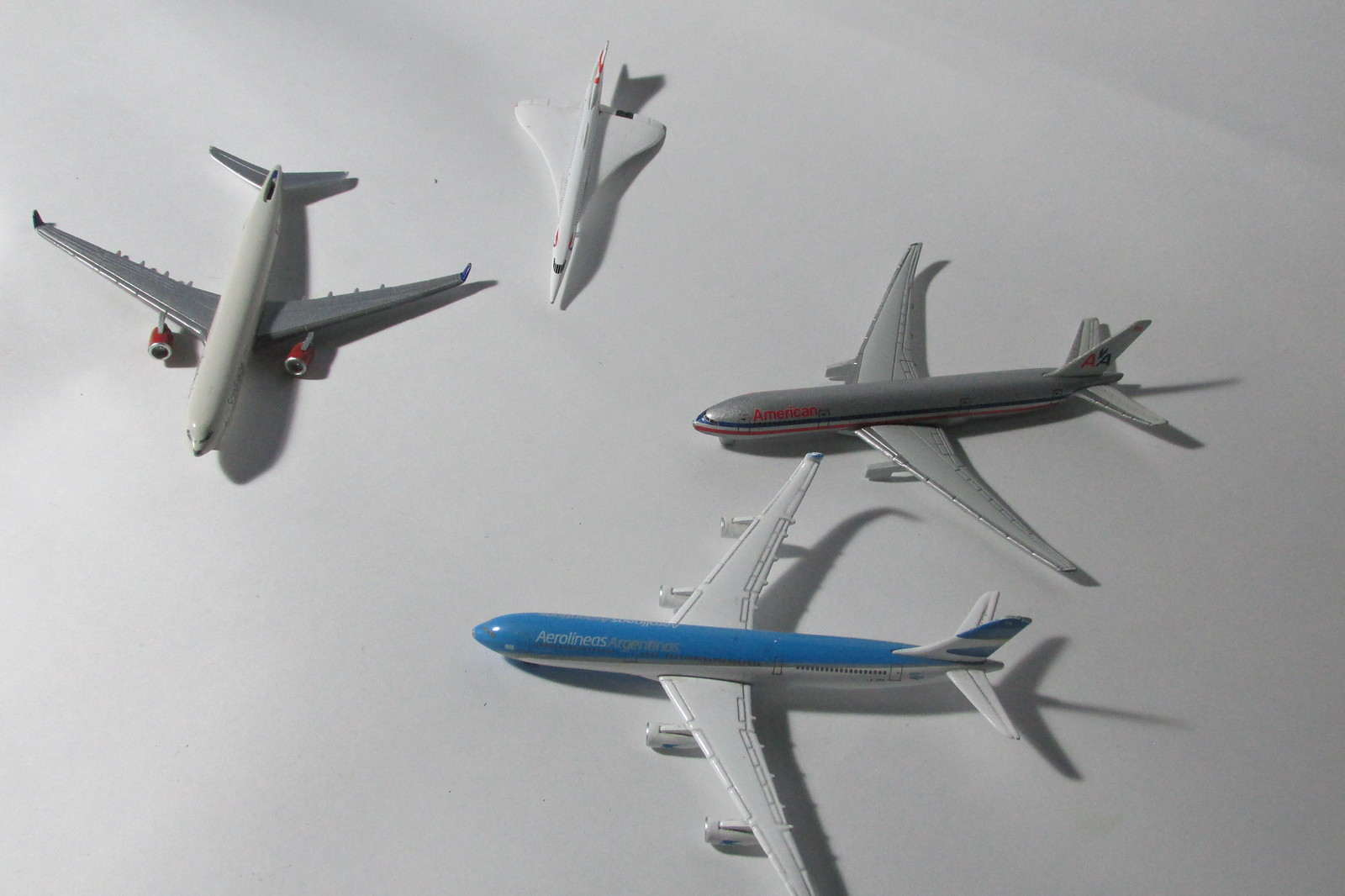The photo features several toy planes, set against a featureless white background which accentuates their distinct shadows. These models predominantly consist of commercial airliners and one unique supersonic transport. Three of the planes are standard passenger jets, while one appears to be a Concorde model, characterized by its sleek white design, highlighting its supersonic nature and differing scale.

Among the commercial jetliners, there are:
1. A silver plane adorned in the American Airlines livery, featuring a red, white, and blue stripe running along its fuselage with "American" written in red on the front and the "AA" logo on its tail.
2. A blue and white aircraft marked with "Aerolineas Argentinas." This model has light blue on its top half with white wings and stabilizers, and it features four white engines, two under each wing. The word "Aerolineas" is written in white on the light blue section, with "Argentina" in a dark gray shade that is less legible.
3. A third jet features gray wings and two underwing engines painted red.

Also present is a white model that appears to be a Concorde, notable for its sleek design, distinguishing it from other conventional aircraft models in the collection. These small models collectively portray an array of aviation history, from typical commercial flights to the iconic, though now-retired, supersonic passenger jet.